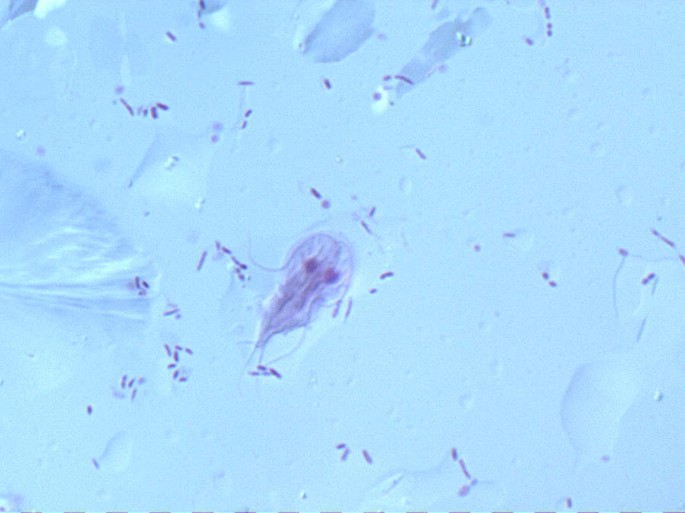The image depicts a microscopic slide with a light blue tint, showcasing a variety of organisms. The central focus is a larger, oval-shaped organism with two prominent black dots that resemble eyes at its head. The creature has hair-like fibers or tentacles at its rear and exhibits a darker blue hue compared to its surroundings. Surrounding this main organism are numerous significantly smaller, oval-shaped organisms, approximately ten times smaller, also in darker blue. These tiny, cell-like organisms appear to be swimming in a watery or plasma-like substance. The overall view resembles a lively scene under a microscope, where the pale blue background is dotted with dark blue specks and shapes, including what looks like a shadowy outline of a leaf on the far left. The scene is filled with intricate details, providing a vivid glimpse into the microscopic world.